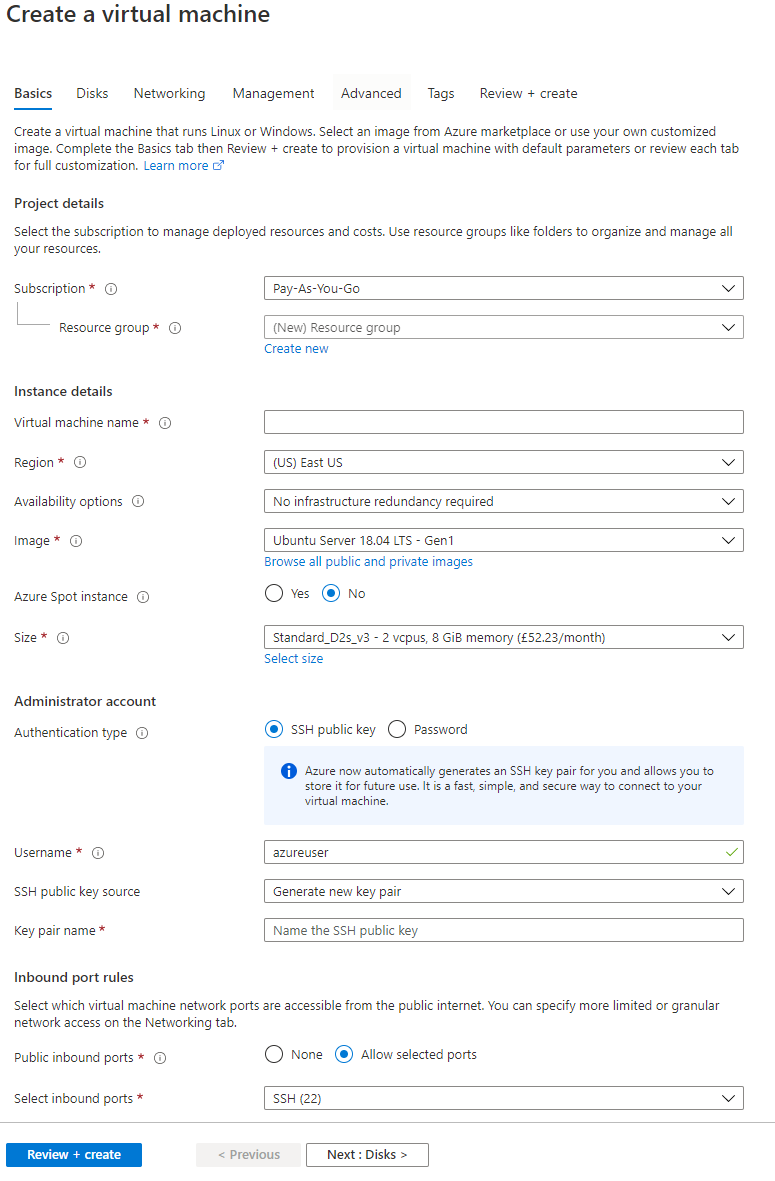**Detailed Caption for Website Image:**

The image depicts the interface for creating a virtual machine on a cloud platform, categorized under "websites." At the top, it prompts the user to "Create a Virtual Machine," followed by an array of tabs: Basics, Disks, Networking, Management, Advanced, Tags, Review + Create. The Basics tab is currently selected.

Below, the interface provides instructions: "Create a virtual machine that runs Linux or Windows. Select an image from Azure Marketplace or use your own customized image. Complete the Basics tab and then click Review + Create to provision a virtual machine with default parameters, or review each tab for customization." 

There is a link for additional information labeled "Learn more."

The form includes fields for selecting a subscription model, with "Pay-As-You-Go" pre-selected, and a field to create or select a resource group, with an option labeled "New Resource Group." User inputs for creating the virtual machine include fields for Virtual Machine Name, Region, Availability, and Image. 

A recording timer noted in the image suggests users are outperforming the expected time for this setup activity, having surpassed both 1:30 and approaching the 2-minute mark, indicating an ongoing recording session without the appearance of a finish recording button.

The interface appears to be stuck, as the timer continues to count, reaching 2:01 and beyond as the finish recording button still hasn't appeared.